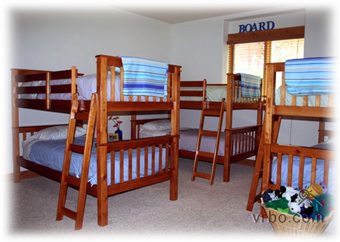This vibrant bedroom, likely a children's room designed for a vacation rental, features three sets of wooden bunk beds with a medium brown stain and bamboo-like frames. Each bunk bed includes a secure ladder and guardrails on the top bunks for safety. The bedding varies across the room, with predominantly blue bedcovers, but also some featuring pink and light plum tones. Draped over the top bunks' edges are striped towels in shades of blue, gray, and white, adding a subtle decorative touch. The room contains a central window framed in wood, topped by the word "BOARD" in large letters. Near one of the beds, there's a basket filled with toys, underscoring the room’s child-friendly appeal. The setting suggests a cozy, shared space, possibly part of a rental property listed on VRBO.com, intended for families vacationing together.